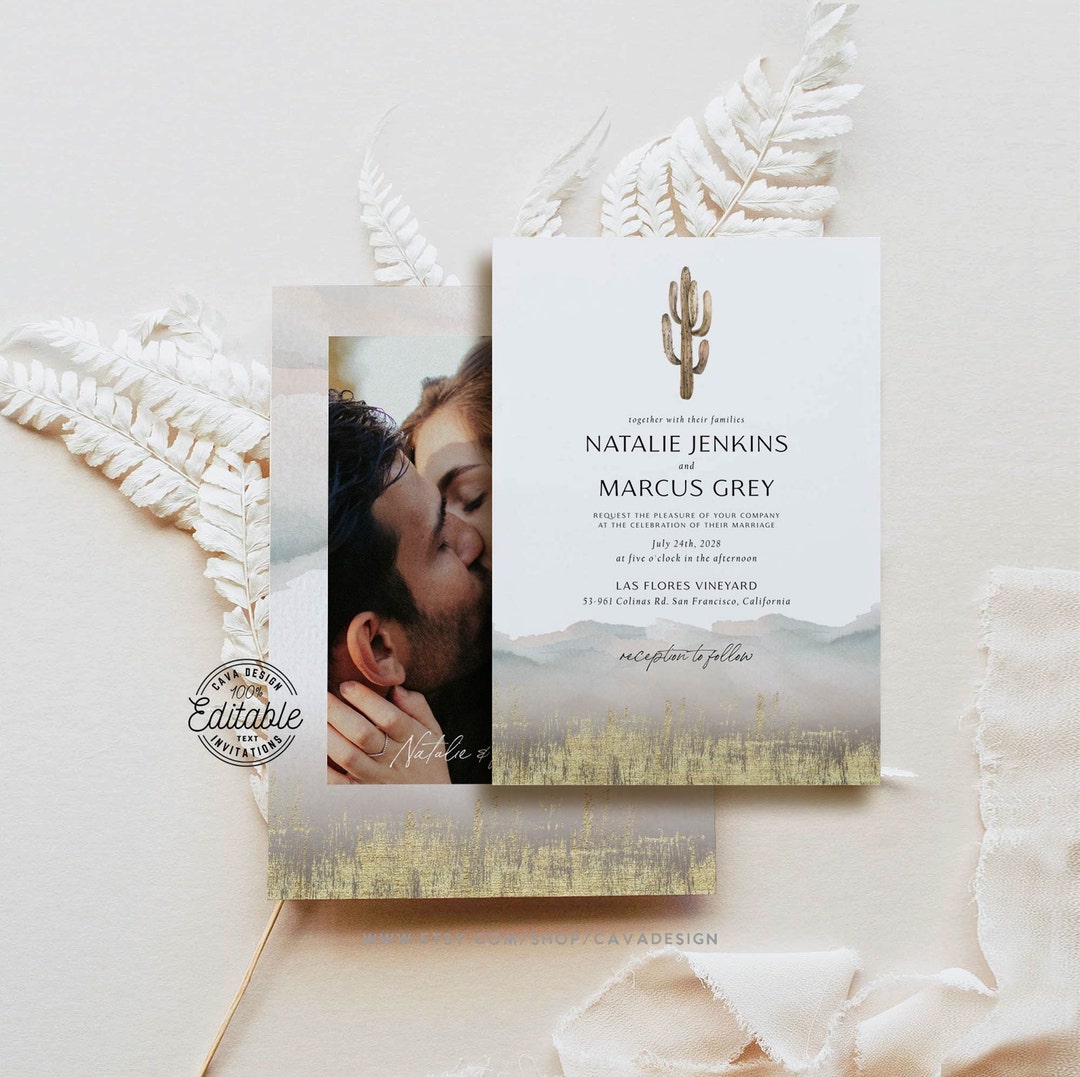The image displays a beautifully designed digital wedding invitation. Set against an off-white backdrop adorned with delicate white fern leaves, the centerpiece of the image is an intricate wedding invitation card. At the top of the card, a green cactus graphic is displayed above the text "Together with their families." The card prominently features the names "Natalie Jenkins" and "Marcus Gray" along with the details, "request the pleasure of your company at the celebration of their marriage," the event date, "July 24th, 2028 at 5 o'clock in the afternoon," and the venue address, "Las Flores Vineyard, 53-961 Culdis Road, San Francisco, California." The bottom of the card includes a cursive script phrase, which appears to be part of a signature or an additional note. 

Adjacent to the invitation text, there is a romantic photograph of a man and a woman sharing a kiss, captured in a tender moment with the woman's hand gently caressing the man's jawline. Her hand, adorned with a ring, emphasizes the intimate nature of the image. To the left of the picture, there is a visible stamp-like design that reads "100% edible, set invitations." Below the central card, in gray text, the words "Kava Design" and other faint, text-related information are printed, adding to the overall elegant and crafted feel of the invitation.